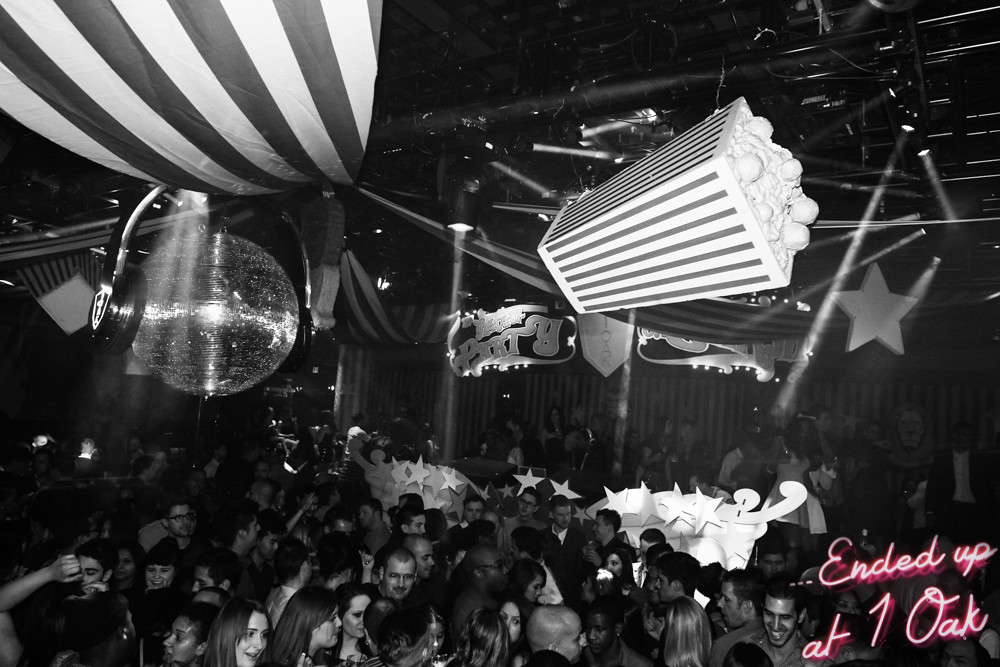This black and white photograph captures a dynamic scene at a bustling nightclub. The image, taken from an elevated perspective, reveals a large crowd of people filling the bottom half, all facing different directions as they enjoy the atmosphere. The crowd is predominantly gathered on the left side of the image. Above them, a large, shiny disco ball adorned with headphones hangs on the left, accompanied by a draped black and white striped tapestry. To the right of the disco ball, a sizeable, horizontally hanging popcorn box, complete with visible kernels, hangs from the ceiling, which itself appears intricate and covered in various contraptions. The center features an elaborate decoration with swirls and colorful five-pointed stars, adding to the festive ambiance. On the right, a prominent five-pointed star is reflected onto a curtain behind the crowd. Lively spotlights beam down onto the partygoers, casting a vivid play of light and shadow. Additionally, the words "party" and "Oak" can be discerned on the wall towards the top, while the bottom right corner features the pink text "ended up at 104."